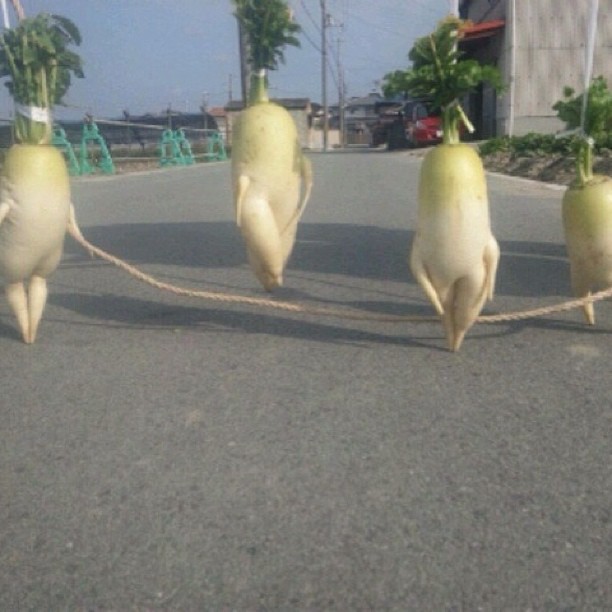This photograph features a cleverly staged scene set on a concrete promenade near a beach, with pine trees and electrical lines visible in the background on a clear day. In the foreground, four large, anthropomorphic daikon radishes are positioned in a playful tableau reminiscent of a jump rope game. Two of the radishes hold the ends of a skipping rope, while the other two wait to jump in. The radishes, which have green stalks facing upwards and various protrusions that resemble human arms and legs, are arranged horizontally across the frame. One of the radishes even appears to have a leg crossed over the other, adding to their unusual, almost human-like appearance. The scene is both whimsical and surreal, capturing a moment of unexpected creativity on a grey concrete road.